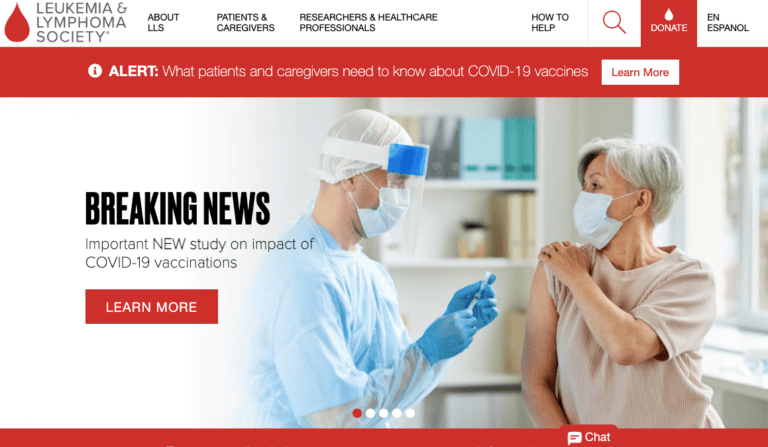This is a detailed screenshot from the Leukemia & Lymphoma Society website. In the top left corner, there's an emblem of a red blood drop adjacent to the "Leukemia & Lymphoma Society" text. Alongside it are the navigation options: "About LLS," "Patients & Caregivers," "Researchers & Healthcare Professionals," and "How to Help." Additionally, there's a magnifying glass icon for search functionality and a prominent red "Donate" button. Users also have the option to switch the website's language to Spanish.

Below this navigation bar, there is an information alert banner addressing what patients and caregivers need to know about COVID-19 vaccines, accompanied by a "Learn More" button. The central image beneath this alert features a healthcare worker in comprehensive Personal Protective Equipment (PPE) – including a hairnet, face shield, face mask, full-body suit, and blue gloves – holding a syringe. Opposite the healthcare worker, a woman seated on a bench or chair has her sleeve rolled up, looking attentively toward the medical professional. This section is highlighted with a "Breaking News" header and details an important new study on the impact of COVID-19 vaccinations.